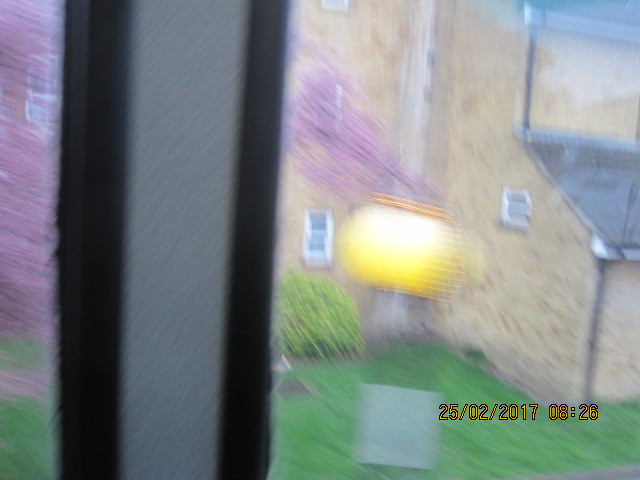The image, taken on February 25, 2017 at 08:26, is very blurry and seems to capture a scene from a window looking out towards a building made of tan-colored bricks. The building is multi-story with a distinctive black roof visible to the right. Above the roof, there's an unusual orange and yellow rounded object, which appears to be levitating near the corner of the building. In the foreground, lush green grass spans the lower part of the image, accented by a large green bush positioned under one of the windows. Additionally, there's a square gray object on the lawn. Despite the blurriness, a purple-like streak or tree branches are noticeable in the image. An orange timestamp in the lower right-hand corner reads "25-02-2017 08:26".